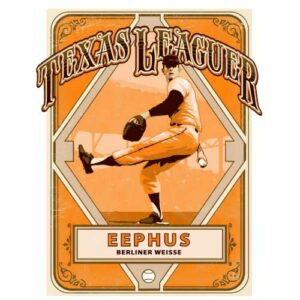The image depicts a graphic design resembling a vintage baseball card. Dominated by an orange background, the card features a diamond-shaped frame in the center showcasing a pitcher mid-throw. The pitcher, balancing on his right leg with his left leg extended forward, is poised with a glove on his left hand and a baseball in his right. The top of the card displays the bold, arching text "Texas Leaguer" in dark brown with a pale cream outline, overlapping the card's background. Below the pitcher, a white rectangle features the text "Eephus Berliner Weisse" in orange. Ornate dark brown curly cues embellish the corners of the card, adding a decorative touch, while a small white baseball design adorns the very bottom. The overall design combines elegance and sports nostalgia, with meticulous attention to detail in its layout.